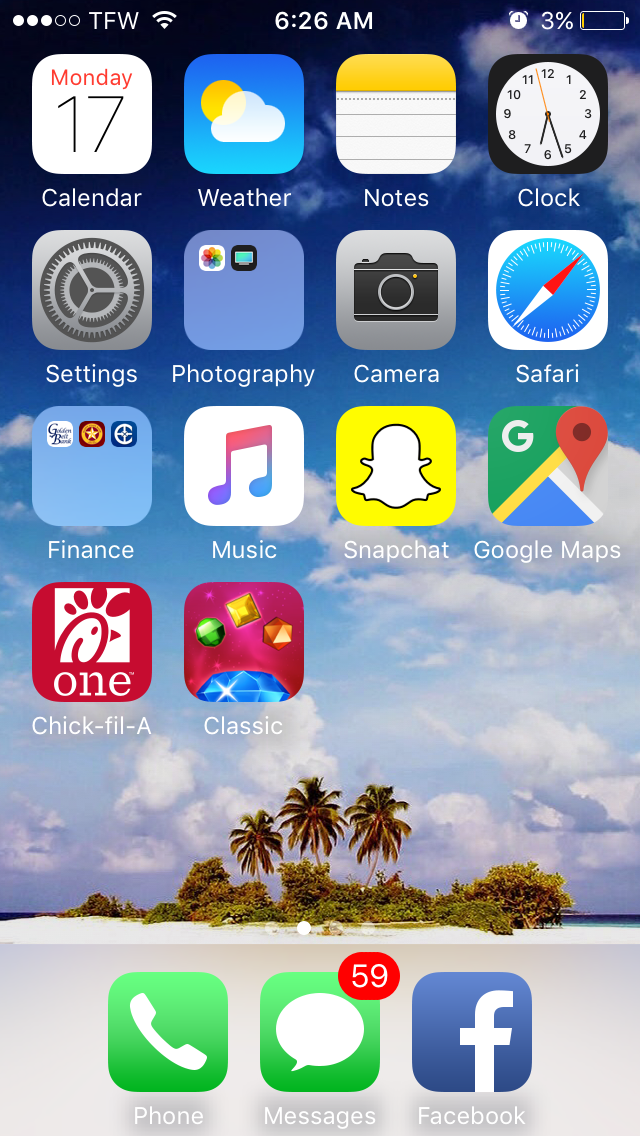This screenshot captures the home screen of an iPhone, identifiable by its distinct icon arrangement and interface design. In the top left corner, the screen shows a cellular signal strength of three out of five bars, accompanied by the carrier label "TFW" in white. Next to this, there's a full-strength, white Wi-Fi icon. The current time displayed is 6:26 a.m., and there is an alarm set. The battery indicator is critically low at 3%, shown in yellow, indicating low power mode.

On the home screen, starting from the top, the first row of apps includes the Calendar app with the date marked as "Monday the 17th," the Weather app, the Notes app, the Clock app, and the Settings app arranged in a tidy column. The following row features apps for Photography, Camera, Safari, and an intriguing array of everyday utility.

Further down, the arrangement extends to include Finance, Music, Snapchat, and Google Maps, followed by another row containing the Chick-fil-A app and a game labeled "Classic." The background image of the home screen depicts a serene island scene, characterized by bright white sand, lush green bushes, and palm trees standing against the backdrop of a blue sky dotted with white clouds.

Finally, at the bottom of the screen, three essential icons are docked: Phone, Messages, and Facebook, providing quick access to communication tools. The overall layout presents a harmonious blend of utility, entertainment, and aesthetics, characteristic of a personalized iPhone home screen.